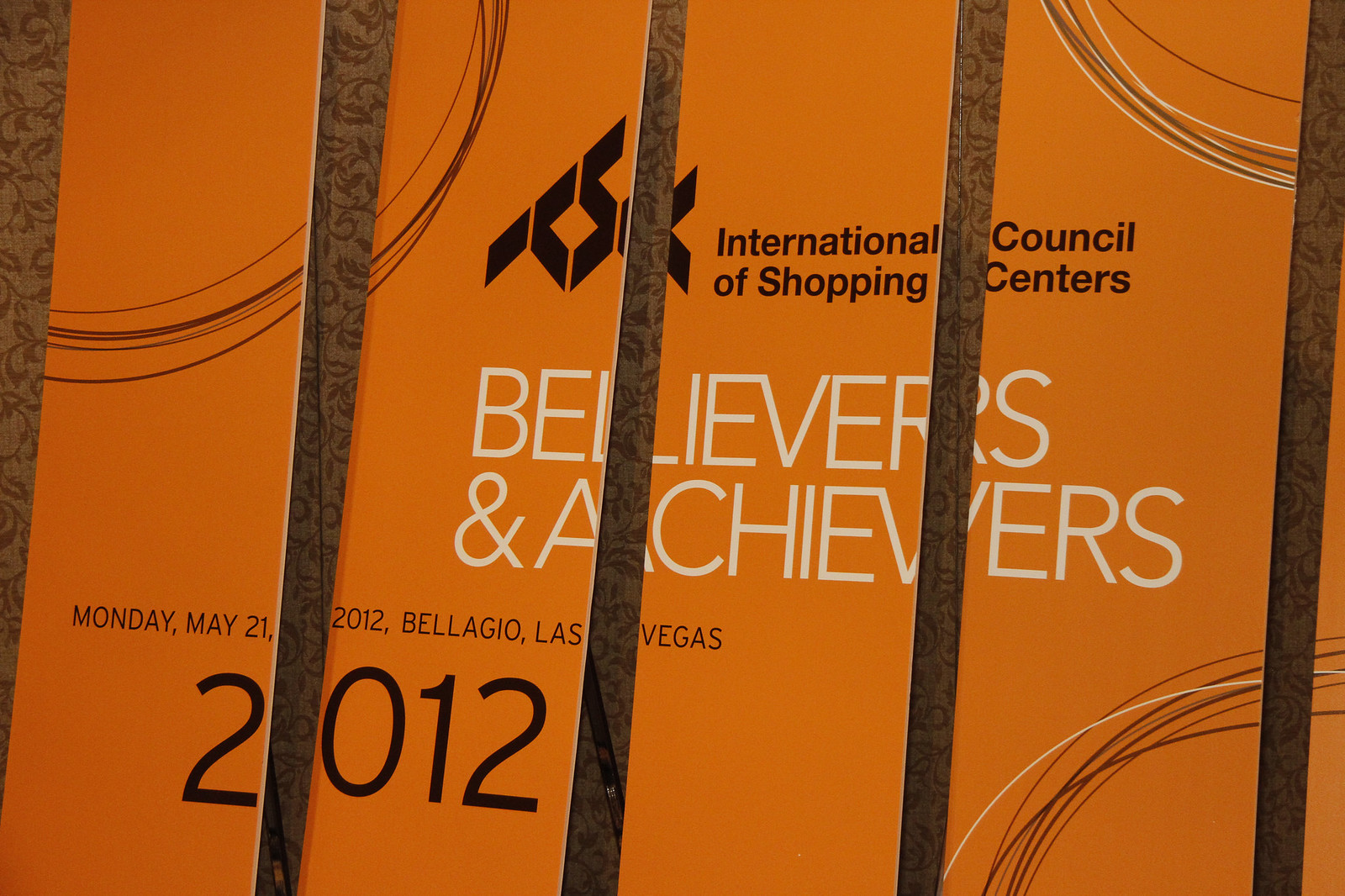This color photograph captures a large segmented sign mounted on a wall, each of its five panels contributing to a unified and legible display. The sign features an orange background adorned with semicircular graphics in the corners and a logo consisting of black geometric shapes. The noticeable text on the sign reads: "International Council of Shopping Centers" followed by "Believers and Achievers" in white text centered in the middle. Additionally, there is black text in the bottom left corner that states: "Monday, May 21, 2012, Bellagio, Las Vegas." The year "2012" is prominently displayed in large black letters, standing out significantly from the rest of the text. The sections of the sign, whether made from metal or wood, are slightly separated but arranged closely enough to maintain clarity.